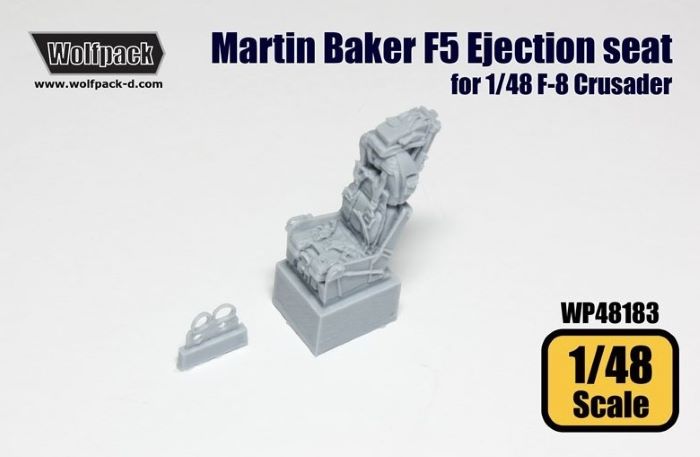This promotional image from Wolfpack advertises a gray, unpainted plastic model of a Martin Baker F-5 Ejection Seat designed for the 1/48 F-8 Crusader. The model is displayed on a flat gray surface with a matching gray background, giving the impression it's floating in a gray void despite its shadows and angled presentation. The top left corner features a gray rectangle with the company logo 'Wolfpack' in gray text with white borders, followed by their website 'www.wolfpack-d.com' in black text beneath it. The top right corner displays blue text reading 'Martin Baker F-5 Ejection Seat for 1/48th F-8 Crusader.' Additionally, in the lower right corner, a yellow rectangle with rounded corners features the black text '1/48 Scale,' with the product code 'WP48183' positioned directly above it.